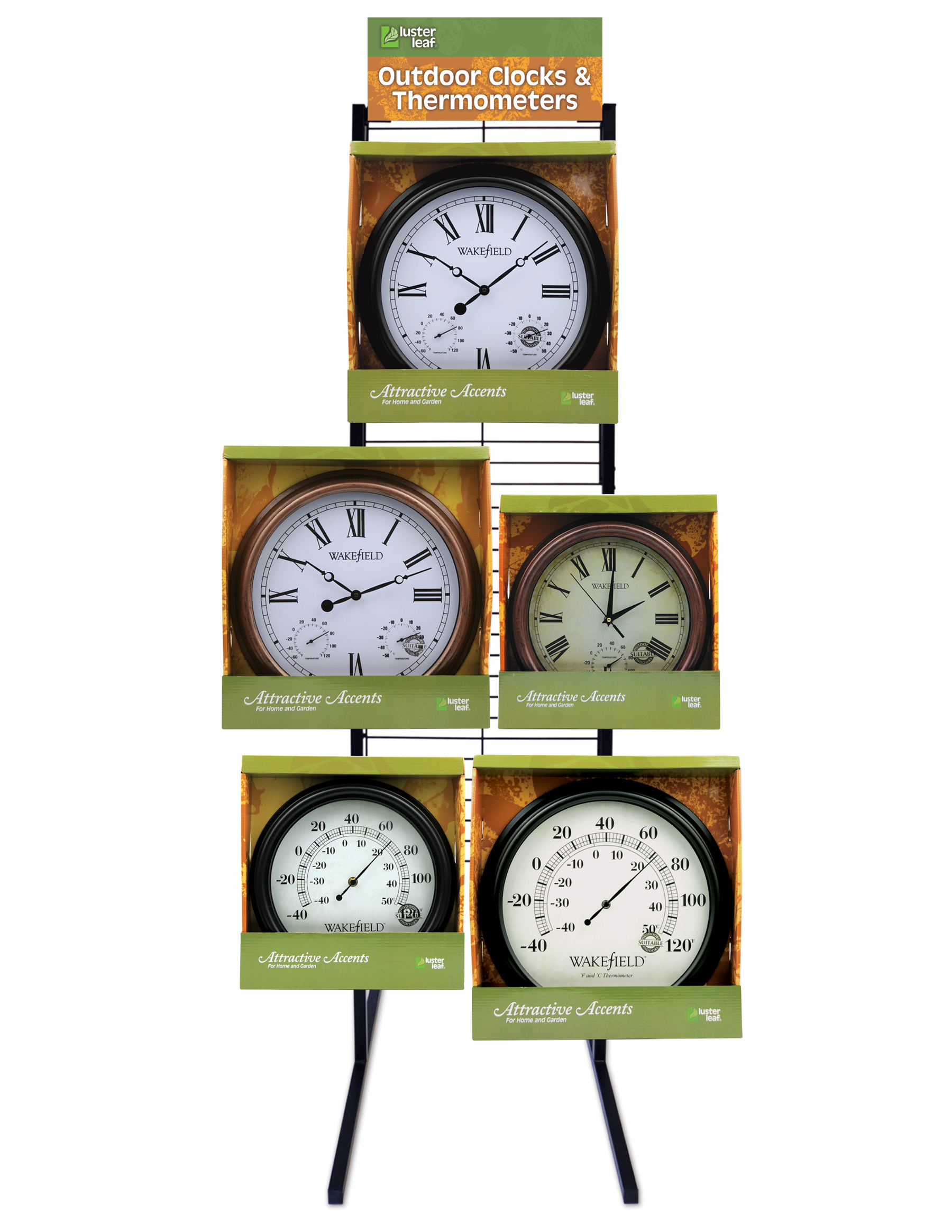This image displays a retail stand featuring five packaged analog outdoor clocks and thermometers. The sturdy black metal frame holds the items visibly, arranged in a single row without any overlapping. A small, green sign at the top, with brown underneath and white font, reads "Outdoor Clocks and Thermometers," indicating the product category. Each clock and thermometer sits within a green cardboard package that has a white background and brown borders, with the brand names Luster Leaf and Wakefield visible.

The top package features a traditional clock with a black frame, white face, black Roman numerals, and black hands, labeled "Wakefield" and "Attractive Accents for Home and Garden." The two clocks directly below are quite similar, displaying slight variations in border color and interior design, with one having a goldish hue.

Below the clocks, the stand showcases two thermometers framed in black, white backgrounds, and numbers ranging from -40 to 120 degrees Fahrenheit. The thermometers are designed in an arch shape, resembling a car's speedometer, and are also branded with "Wakefield." The overall backdrop of the image is white, providing a clear, unobstructed view of the display stand and its contents.